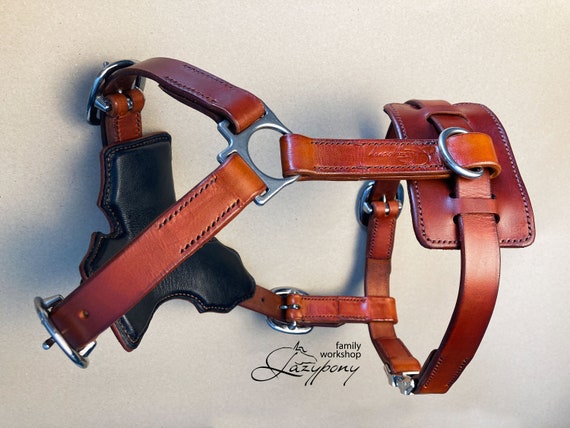The image showcases a brown leather harness that appears to be designed for medium-sized animals, possibly a dog or a small horse. The leather has a reddish tint reminiscent of cherry wood, with black leather accents on the left side. Notable features include silver metal belt hooks and a strap with a notch for fastening. One end of the harness has a loop for attaching a leash. Beneath the harness, the text "Family Workshop Lazy Pony" is displayed, with "Family Workshop" in a sans-serif font similar to Calibri and "Lazy Pony" in a cursive font. The background of the image is primarily ivory, though it has been described as gray in one instance. This detailed and curious contraption could easily serve various small animals.